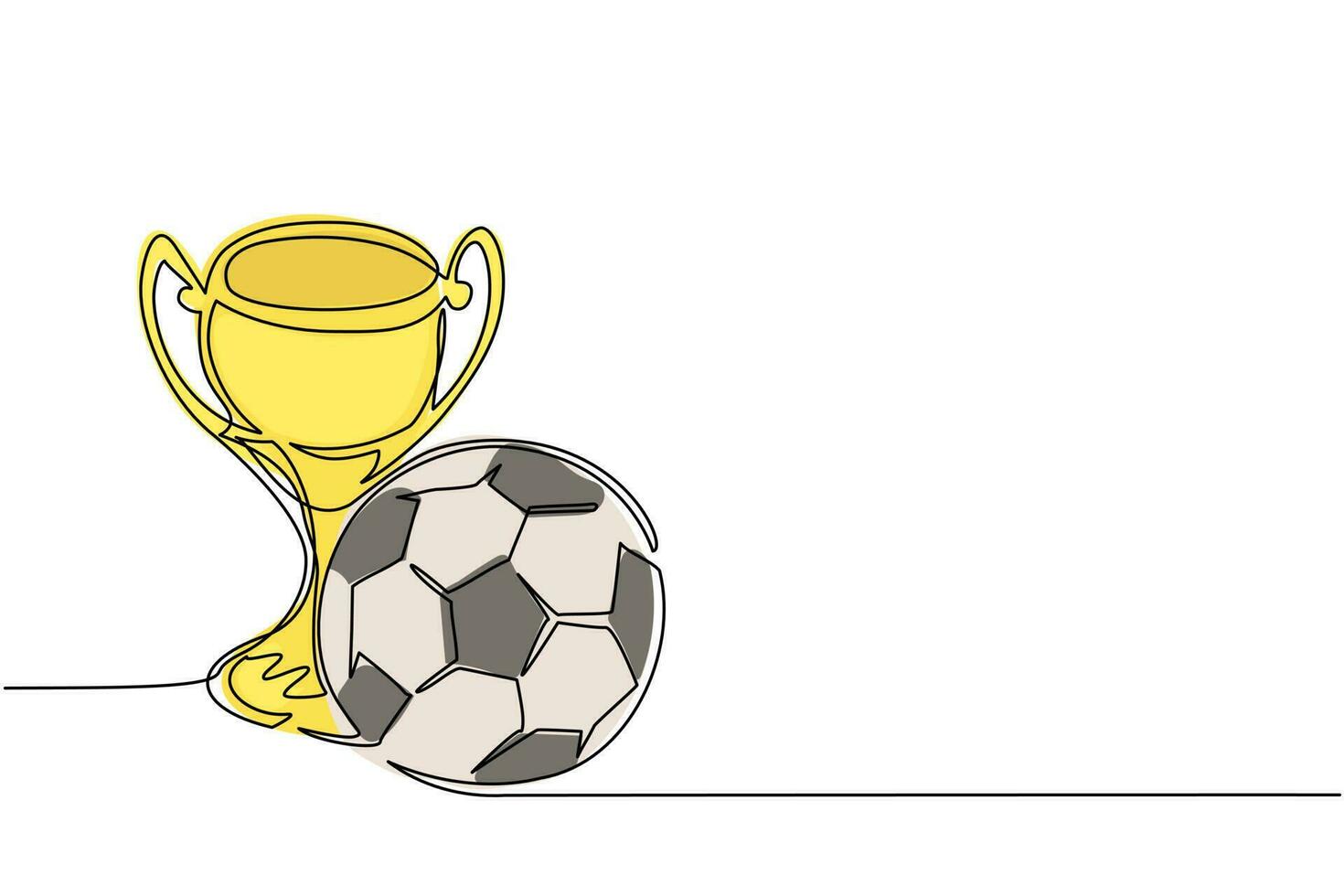This is a minimalistic, hand-drawn graphic depicting a gold trophy cup and a soccer ball composed of off-white and gray pentagons. Set against a white background, the drawing utilizes continuous black lines to create a cohesive visual. Positioned on the left side, the trophy features a prominent round bowl with two ornate handles, tapering into a long cylindrical stem with a round base. On the right, in front of the trophy, sits a soccer ball, characterized by its polygonal pattern. The lines seamlessly connect the elements: one horizontal line extends from the left edge, passes through the trophy, then wraps around the soccer ball before continuing to the right edge. The design invokes simplicity, akin to illustrations found in children's books, emphasizing the themes of soccer and accomplishment.